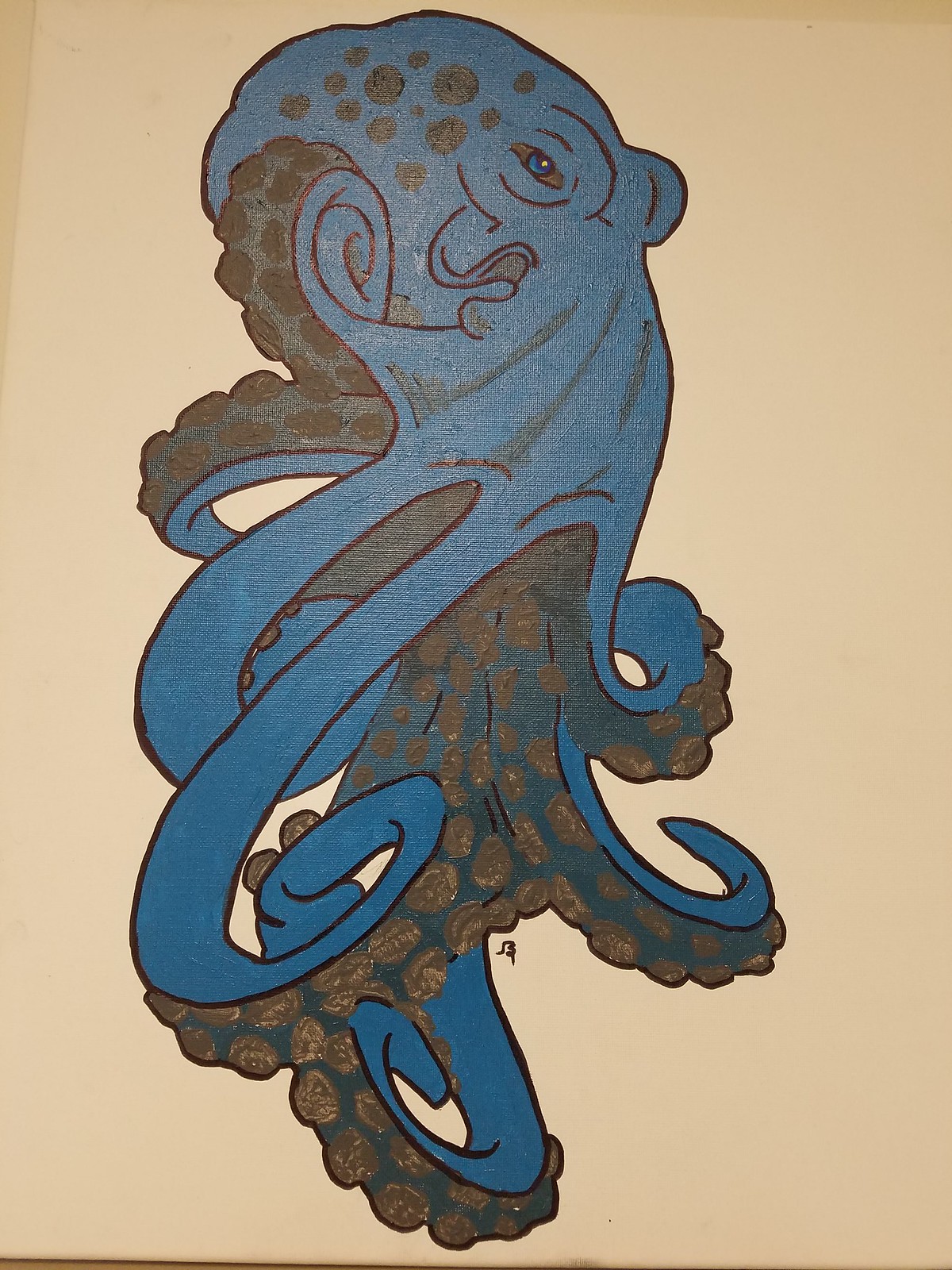This image features a simple yet charming drawing set against a light dusty pink background. The artwork appears to be created using colored pencils or ink, showcasing a stylized and somewhat cartoonish rendition of an octopus. The octopus itself is rendered in a slate blue hue, with its head positioned at the top of the composition. The tentacles are depicted in varying shades of gray on the underside, adorned with goldish-colored knobs. These tentacles are intricately coiled, adding an element of dynamic movement to the piece. The overall design is both whimsical and detailed, enhancing the playful nature of the illustration.